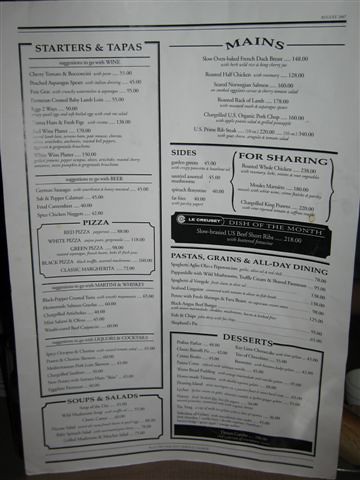The image captures a photograph of a restaurant menu, presented on a long, white rectangular piece of paper with black font. Although the picture is slightly blurry, making it difficult to read the specific dishes, the main section titles are discernible. At the very top, a black line stretches across the menu, delineating the sections. The first section, labeled "Starters and Tapas," lists various items along with their prices, though the individual names are unclear due to the blur.

In the middle of the menu, a dedicated section for "Pizza" enumerates different types of pizzas, each accompanied by their respective prices. Moving down to the bottom left corner, the "Soups and Salads" section is visible. On the top right, another section labeled "Mains" appears, and directly underneath, there are two smaller sub-sections titled "Sides" on the left and "For Sharing" on the right.

Further down, a segment for "Pastas, Grains, and All-Day Dining" is visible, listing various options with corresponding price tags. The bottom right-hand corner features a section outlined in a black rectangular box, titled "Desserts," which again lists different dessert options along with their prices. Despite the blur, the structured layout of the menu is clear, with each section thoughtfully organized to guide diners through the variety of culinary offerings.